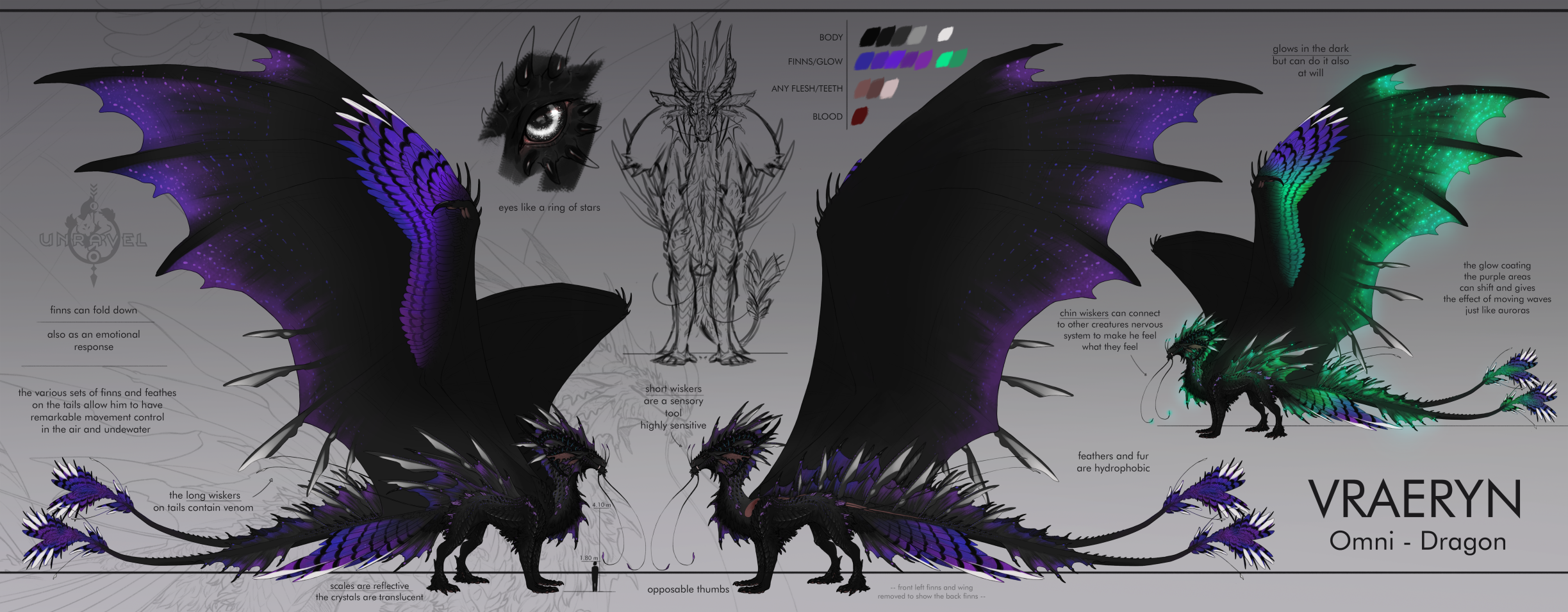The image is a long, thin, horizontal chart with a light gray background. On the far left, there is a colored illustration of a dark, possibly black or purple, dragon facing right. This dragon has large wings extending up and to the left, with some blue coloring and white tips on the right side of the wings. The dragon has white markings on its backside, head, and sides. It has a tail that diverges into two ends. To the left of its wings, there is black writing and a symbol, and to the right of its wings is another symbol and a diagram of a standing dragon facing forward.

In the center of the chart is another dark (either black or purple) dragon, similar in appearance to the left one, but it is facing left and lacks the blue parts of its wings. Above its wings is some black text, and to the left of the top of its wings are color splotches with black writing beside them.

On the far right is a smaller, green dragon facing left, with black writing above and to the right of its wings. In the bottom right corner of the image, there is black text that reads "VRAERYN" in capital letters, and underneath it in smaller print, "Omni-Dragon." The background contains various texts and symbols not easily readable, and at the top of the image, there is a depiction of a dragon's eyeball, presented in a sketch art style. This chart seems to serve as a reference page for different dragon designs.